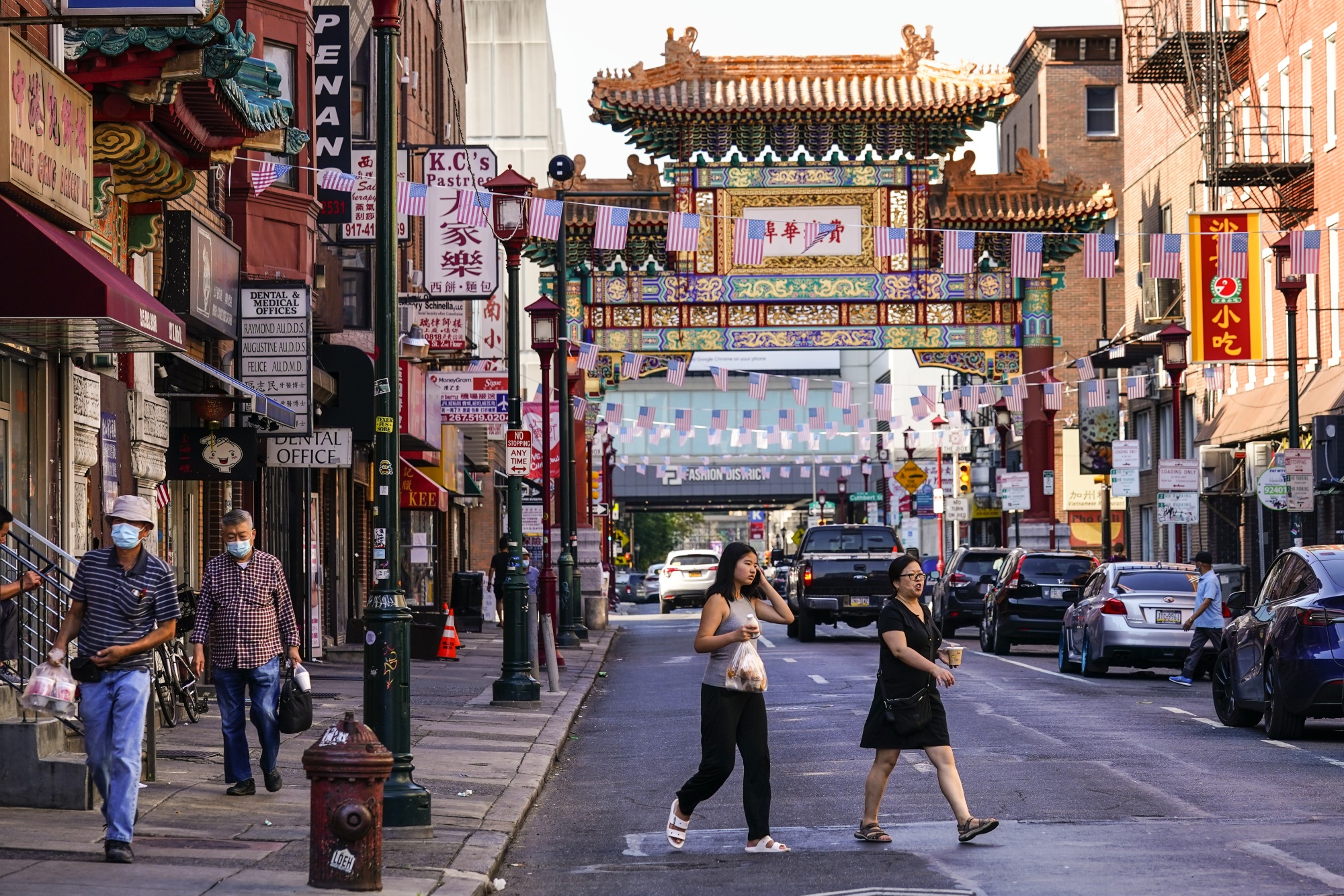This detailed color photograph captures a bustling street scene, likely in a Chinatown district within the U.S.A., characterized by its blend of American and Asian cultural elements. The image shows an asphalt street with concrete sidewalks lined with lampposts and Chinese lanterns. A string of American flags hangs across the top of the street, adding a festive touch. In the foreground, two women are seen crossing the street, which appears to have two to three lanes of one-way traffic moving away from the viewer. Parallel parked cars line the buildings on either side.

On the left side of the image, two men wearing blue face masks walk down the sidewalk, one carrying a clear bag filled with what seems to be takeout Chinese food. Storefronts with signs in both Chinese and English are visible, including "Casey's Pastries" and "Dental and Medical Offices." The street is adorned with Asian-inspired elements, such as an elaborate pagoda-style gateway with a golden roof, which serves as an eye-catching centerpiece. High above in the background, a large overpass can be seen, under a light white sky that accentuates the urban ambiance.